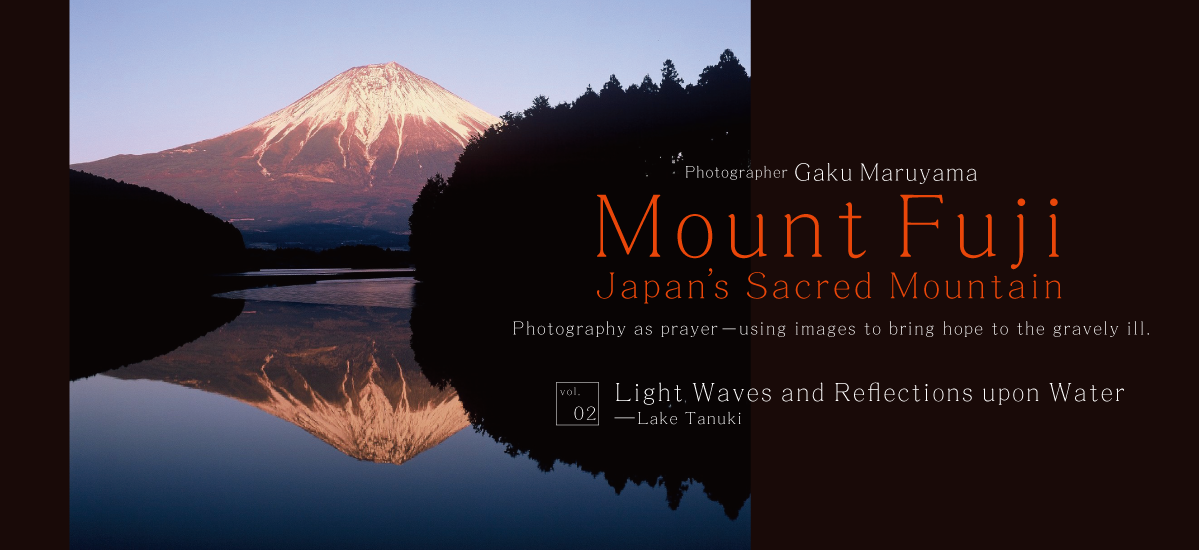The image, a long horizontal rectangle, captures a breathtaking photograph of Mount Fuji, the iconic snow-capped mountain, under a clear blue sky. The serene waters of Lake Tanuki below reflect the mountain with mirror-like precision, creating a mesmerizing double image. Framing the mountain on either side are dark clusters of trees, their forms also mirrored in the still lake. Against a dark black background, bold red text highlights key details: "Mount Fuji, Japan's Sacred Mountain." Above this, it reads "Photographer: Gaku Maruyama," and further below, "Photography as Prayer, Using Images to Bring Hope to the Gravely Ill." The title "Light Waves and Reflections Upon Water at Lake Tanuki" encapsulates the essence of the photograph, which is not only visually striking but also deeply evocative, intended to inspire and offer solace.